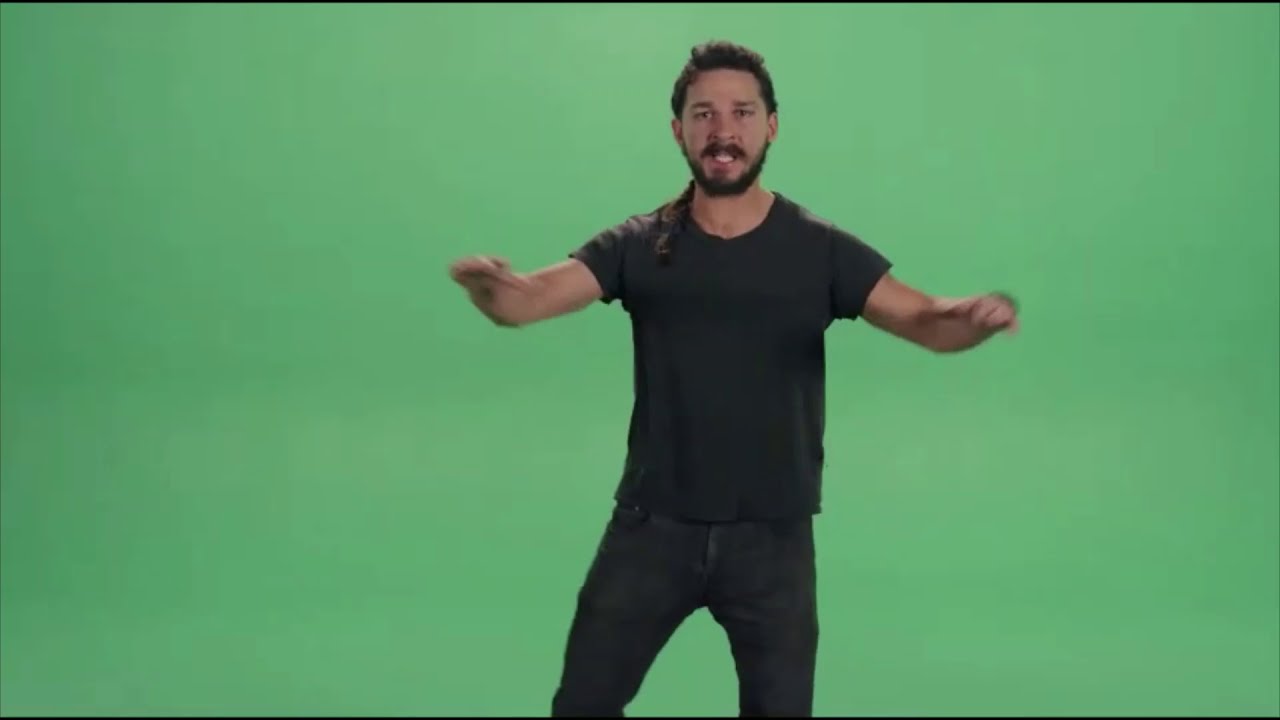The image features actor Shia LaBeouf standing against a distinctive green background that resembles a green screen, typically used for creating memes or GIFs. The photo, which is rectangular and measures approximately six inches wide by three inches high, also includes a thin pinstripe border at the top and bottom. Shia LaBeouf is captured from the knees up, positioned directly in the center of the frame. He is of Caucasian descent, with short curly brown hair pulled back into a ponytail that drapes over his right shoulder. His facial hair consists of a thick brown mustache and beard. LaBeouf appears to be angrily shouting, his mouth open, revealing some teeth. His arms are bent at the elbows and extended forward, as if he’s gripping an invisible motorcycle's handlebars. He is dressed casually in a gray short-sleeved crew neck t-shirt paired with gray jeans. The background is a vivid, uniform green, suggesting the intent to overlay other images or text behind him in post-production.